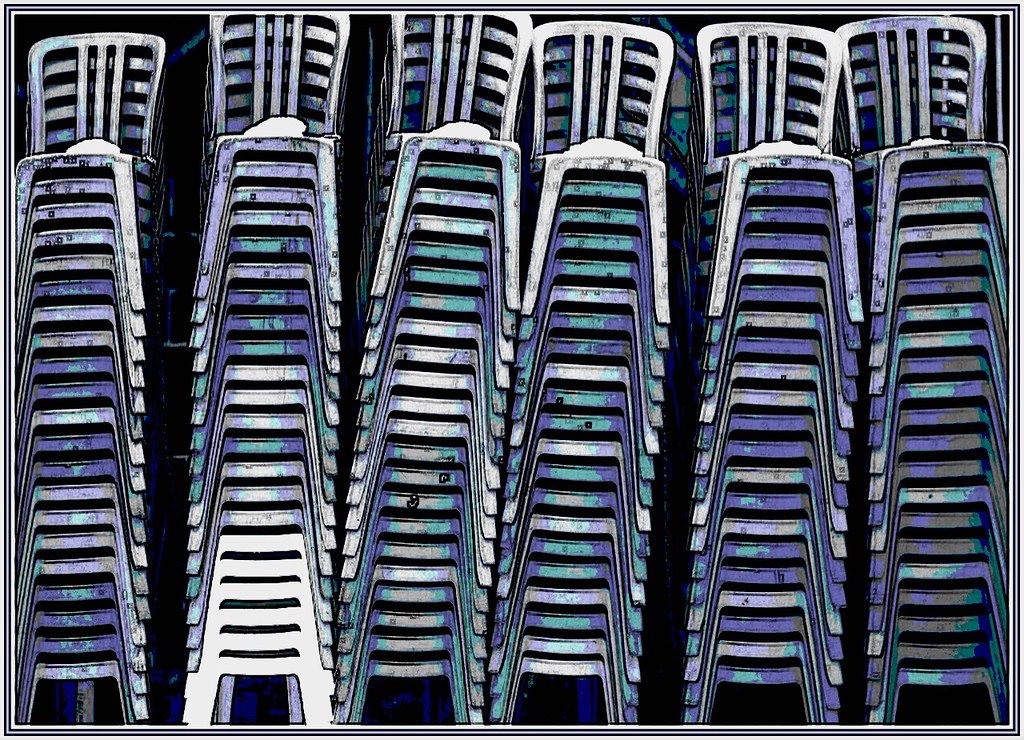The image depicts six closely placed stacks of plastic lawn chairs, each piled in varying heights, with some stacks reaching around 20 chairs. The chairs are predominantly white, though many have splashes of purple, teal, blue, and green, giving each stack a unique and somewhat weathered appearance. The scene, which has a digital or heavily manipulated photographic quality, is devoid of any other elements, set against a dark, black background that provides no scale reference. The chairs, which feature a plain design with three vertical slats on the backrest and additional perpendicular supports, create an intricate pattern of lines and shapes. The colorful, aged look of the chairs suggests they might have been exposed to the elements, adding to their varied palette and somewhat faded look. The overall composition resembles an art print or a drawing, emphasizing the artistic nature of the arrangement.